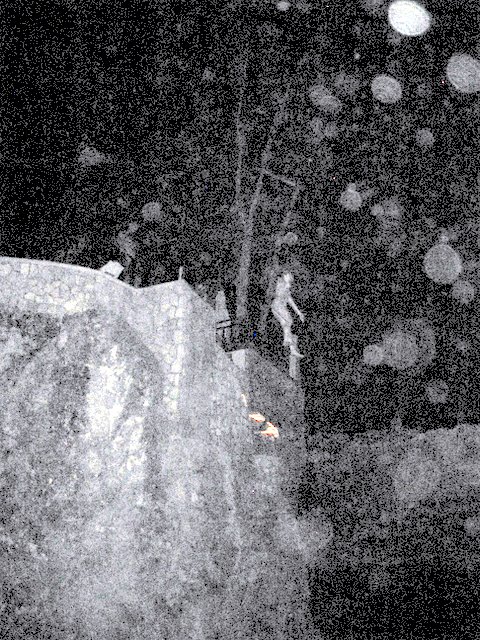The image is a very blurry and grainy black-and-white photograph, possibly a color photograph of a black-and-white image, which adds a slight brownish tinge to certain areas. The photograph appears highly out of focus and grainy, giving it an impressionistic feel. 

Dominating the composition is what looks like a wall made of irregularly shaped stones, which transitions from a curved form to a more rectangular shape. This wall, although composed of stones, appears smooth in texture. The scene is situated on a cliffside, creating a stark contrast between the man-made structure and the natural backdrop. 

In the center of the image, there is a faint, almost indistinct figure of a woman. Her form includes visible details of her head, shoulders, and torso. Beside her, to the left, there seems to be an object resembling a basket. The area to her left is a large pale grey space, enhancing the cliffside impression. Just behind her and to the right, the photograph darkens, filled with numerous small blobs, possibly hinting at a snowstorm or simply adding to the visual noise created by the grainy quality of the image. 

At the top center of the image, there's a distinctive bright red line or triangle, suggesting possible thermal imagery, which stands out sharply against the monochromatic tones.